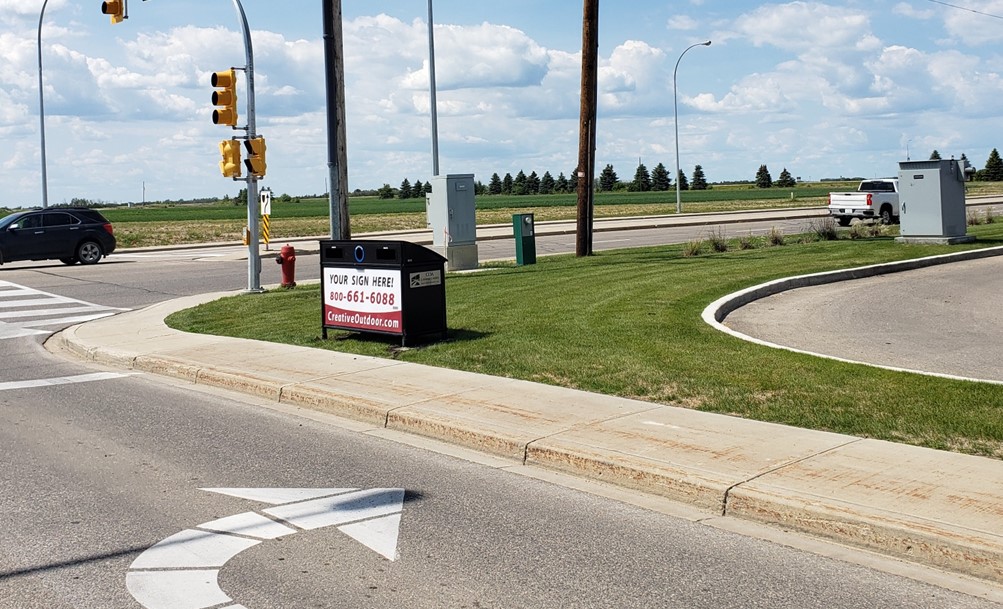In this daytime image, a clear blue sky with white clouds stretches across the top, illuminating the scene with bright sunlight. The central focus is a curved road featuring white markings, including lines and directional arrows. On the road, a black SUV and a white pickup truck navigate through the intersection, the latter appearing to make a recent turn. Surrounding the road are several elements of urban infrastructure: yellow traffic lights, streetlights, electric poles, and a fire hydrant at the corner. A pavement with a pedestrian crossing runs alongside, bordered on its other side by a lush green grassy area dotted with an electrical box and a black desk-like structure displaying a sign that reads, "Your Sign Here, 800-661-6088, creativeoutdoor.com." In the far background, a large green field filled with trees adds a touch of nature to the urban landscape.